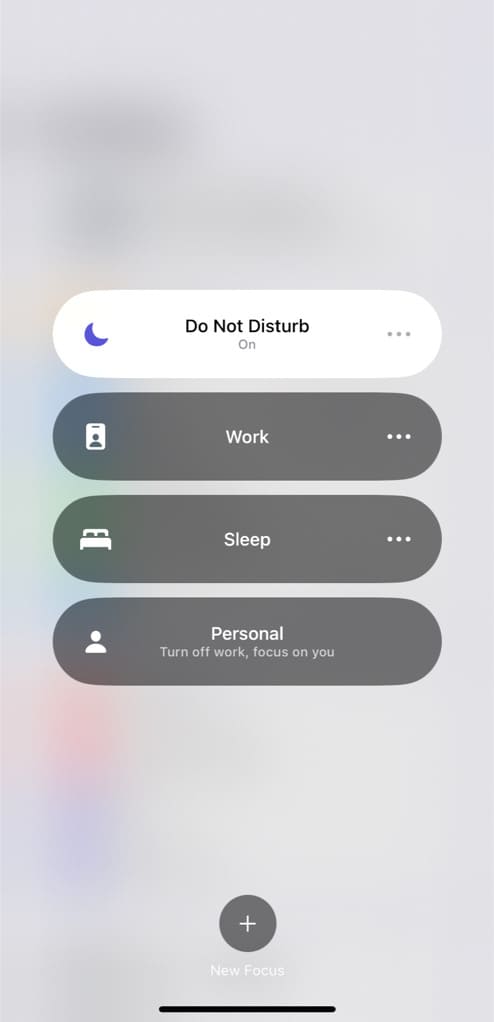The image depicted is a vertically elongated cell phone screenshot, approximately three times taller than it is wide. The entire background of the screenshot is heavily blurred with a gray overlay, rendering it nearly opaque. What can be discerned through the blurred background are vague blobs of color: a yellow square appearing about one-third down the left side, followed by a blue square, green, purple, red, and finally, dark purple, extending to about the halfway mark of the image's height.

Overlaid on top of this background, starting around the one-third mark, is a series of buttons. The most prominent button is the "Do Not Disturb" button, easily identifiable by its yellow outline and moon icon on the left side. This button is currently selected, indicated by its white background. Below it, three additional, equivalently sized buttons are stacked: 

1. **Work** - Featuring a dark gray background with white text and a building icon on the left side. It includes three dots on the right, likely suggesting more options.
2. **Sleep** - Displaying a bed icon on the left side and similar three dots on the right, this button shares the same dark gray background with white text.
3. **Personal** - Showcasing a small person icon on the left side with the same background and text style as the previous buttons.

Beneath these primary options, a dark gray section reads "Turn off at work, focus on you." At the very bottom of the image is a distinct gray circle featuring a white plus sign, likely a button for adding new options or settings.